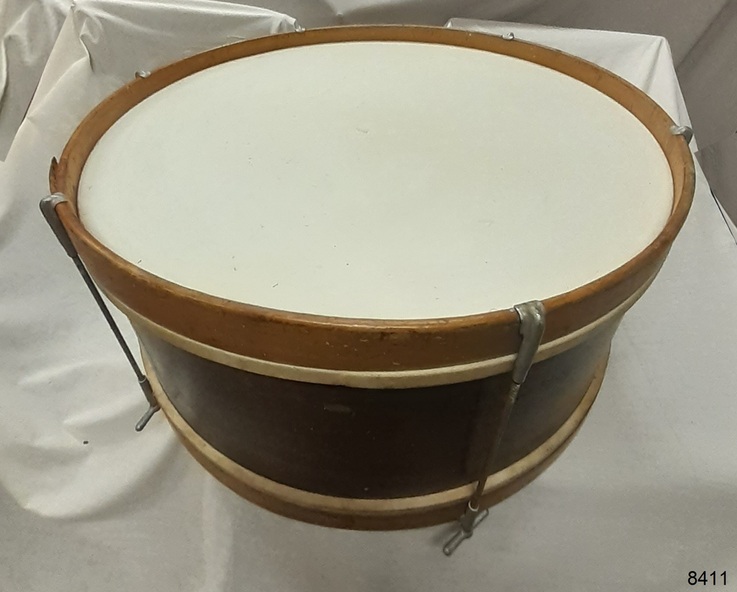The image depicts a large, old-fashioned bass drum positioned on a white cloth or sheet. The drum has an off-white surface top where it is struck, and this is encircled by a mid-grade brown wooden exterior that appears slightly faded and scratched. The edge of the drum is black, and six metal hooks are affixed to the wooden sides, providing connections that resemble hose bibs. In the center of the drum's exterior, a light brown section stands out from the surrounding wood, bordered by a dark brown or nearly black area. In the lower right corner of the image, the numbers "8411" are prominently displayed in black font, while the background in the top right corner of the image is notably bright.